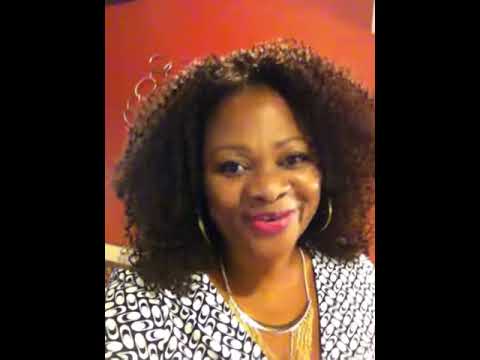The image depicts an African-American woman shown from the sternum up against a red-orange background, likely a wall. She is smiling and appears to be talking directly to the camera, suggesting she might be filming a selfie video. Her shoulder-length hair is curly and slightly poofed at the top and sides. She is wearing pink lipstick and hoop earrings. Around her neck is a semi-circle pendant necklace with dangling gold chains. She dons a black and white patterned suit jacket or blouse. The image quality seems slightly pixelated, possibly due to streaming, and it is framed with two large wide bars on either side, occupying about 20-30% of the total space, leaving no additional context or information about the location.